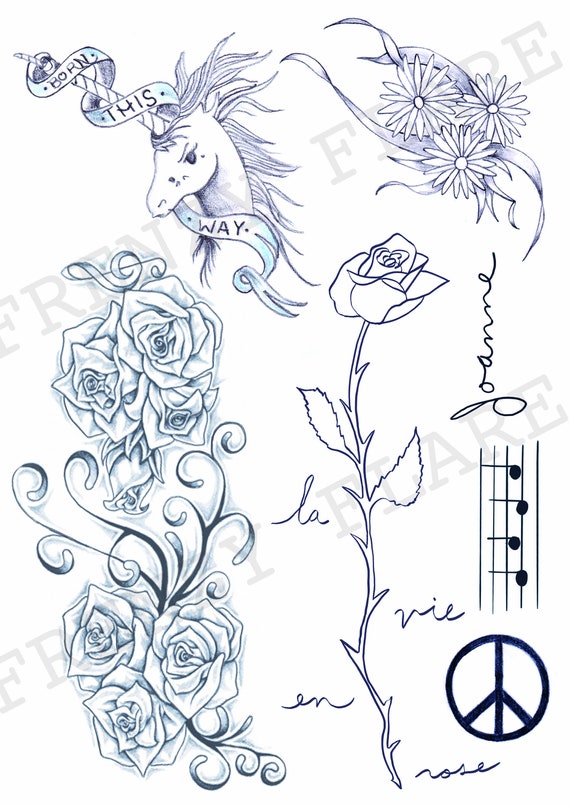The image is a monochrome series of detailed pencil-style drawings on a dense white sheet of paper. In the top left corner, there is a unicorn adorned with a banner reading "Born This Way" wrapped around its horn. Adjacent to it in the top right corner are three daisies, each with ribbons hanging beneath them. Below the daisies and towards the center-right of the image is a peace sign, and to its left, the words "La Vie en Rose" flank a single long-stem rose. Directly to the right of the rose, a musical staff with notes intersects the word "Joanne" written vertically. Additionally, to the left of this central rose, there is a cluster of six roses surrounded by swirling lines. Faintly visible across the image, the watermark "Frenzy Flair" is seen, stretching diagonally from the middle left to the upper right, and reappearing from the lower right to the center right of the image.